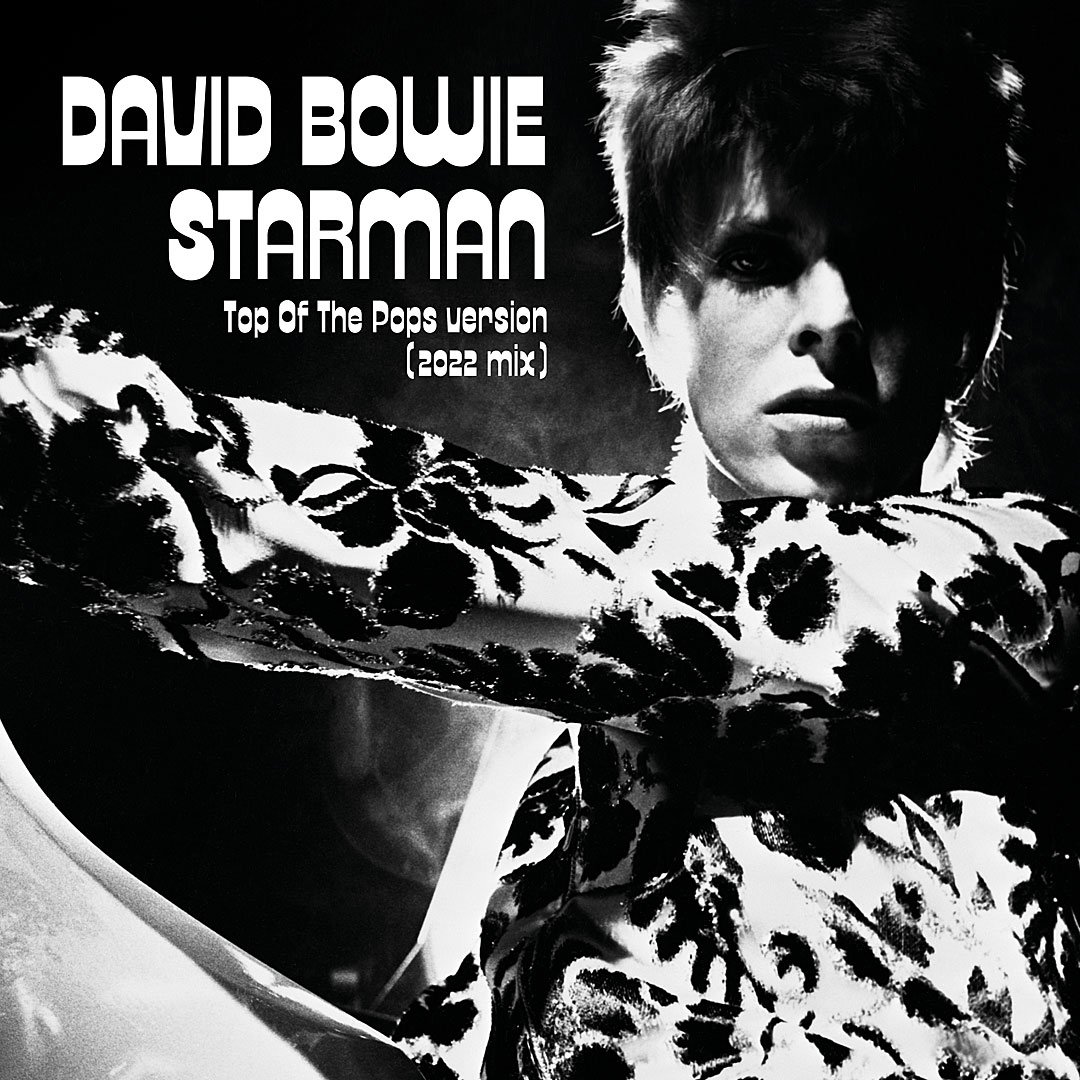This is a black and white cover of a CD featuring a young David Bowie, likely taken in the 1970s. The background is predominantly black with a slightly gray gradient caused by stage lighting shining above his shoulder. Bowie, who appears to be in his early twenties, is dressed in a striking black and white floral-patterned, sequined shirt. His left arm is extended out in front while holding a guitar. His partially lit face, overexposed ear, and long hair create a dramatic look, with his eyes gazing forward and mouth slightly open. In the top left corner, bold white letters state: "David Bowie, Starman, Top of the Pops version (2022 Mix)." The image captures both the elegance and intensity of Bowie during his early career, giving it a distinct, almost glowing effect against the dark backdrop.